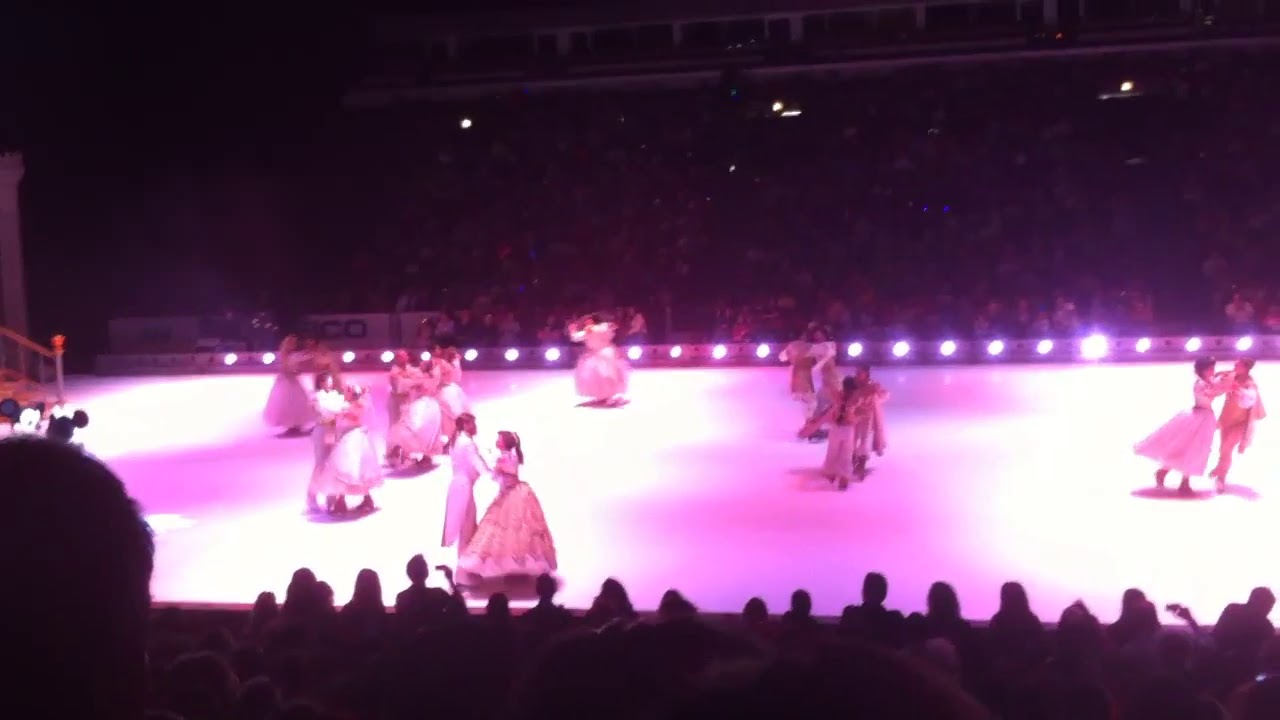The image captures a vibrant indoor ice-skating performance, likely a Disney on Ice show, set within a large arena. Couples, consisting of men and women, elegantly glide and dance on the white ice rink. The women predominantly wear dresses, while the men don more formal attire, reminiscent of 18th-century costumes with long jackets. Bright and colorful lights, including purples and whites, illuminate the rink and enhance the festive atmosphere. Silhouetted spectators surround the rink, attentively watching the performance from the stadium seats on either side. To the left side of the scene, a detailed set design, including recognizable Mickey Mouse characters in costume, adds to the show's thematic elements. A staircase with gold and silver railings is also visible, providing access to the rink. The audience members remain in shadow, highlighting the performers on the ice.